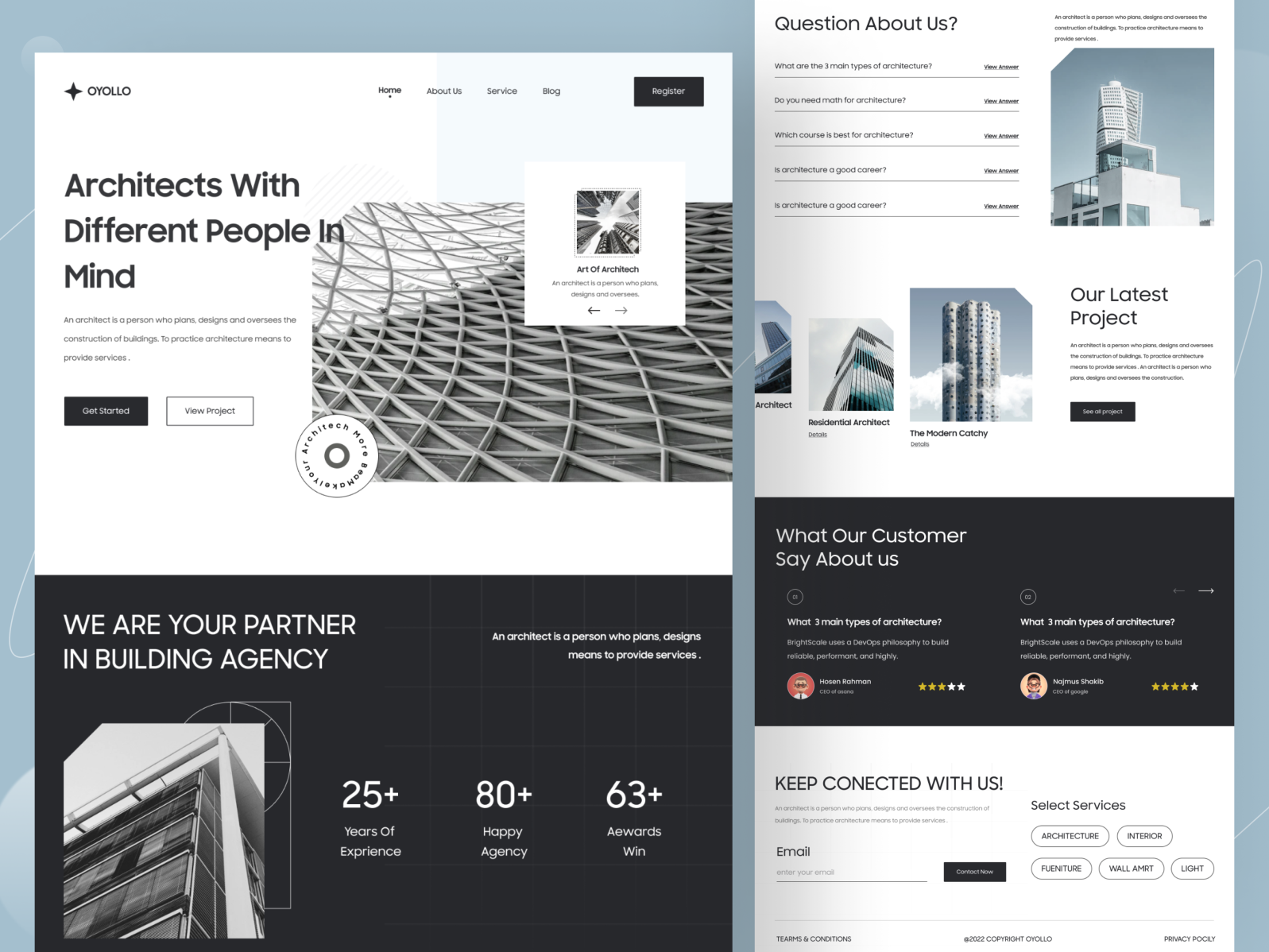The image features a UI design for a website called "OYOLLO." The top left corner displays the company name "OYOLLO," while the main navigation menu in the middle includes links to Home, About, Service, Blog, and a Register button on the right.

Beneath this menu, a tagline reads "Architects with different people in mind," accompanied by a brief description: "An architect is a person who plans, designs, and oversees the construction of buildings. To practice architecture means to provide these services."

This section also includes two call-to-action buttons: a black "Get Started" button and a white "View Project" button. The hero image showcases an interior view resembling the Louvre, with glass triangular structures and an overlay text that includes "Architect." The word following it is partially upside down and unclear.

Below this, there's a section with navigational tools labeled "The Architect, Architecture," and some descriptive text about architects. Arrows at the bottom allow users to browse more photos. 

The lower part of the page highlights the company's credentials and achievements, stating, "We are your partner in building agency," with over 25 years of experience, more than 80 happy agents, and 65 awards won. 

A corresponding side panel presents FAQs including: "What are the three main types of architecture?" "Do you need math for architecture?" "Which course is best for architecture?" "Is architecture a good career?" and a section featuring customer testimonials with a prompt to "Keep connecting with us."